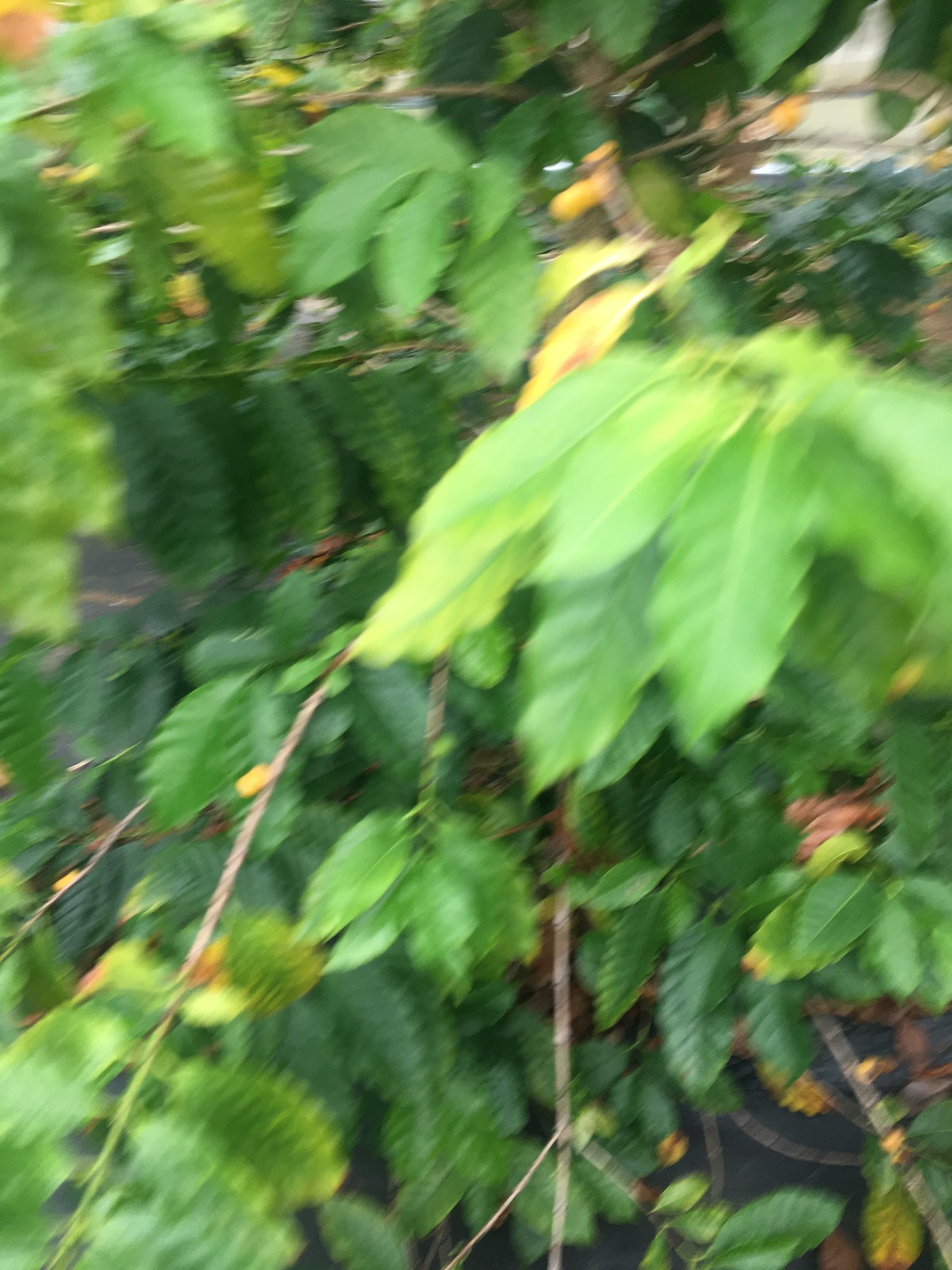A slightly blurry daytime outdoor photograph captures an intimate view of a leafy green plant. The image, though somewhat obscured by motion blur, reveals an array of leaves in varying shades of green, with some appearing darker than others. Veining in the leaves is visible, adding texture and depth to the scene. Scattered amongst the foliage are brown twigs and patches of brown soil. The plant appears to be adorned with circular yellow objects, possibly flowers or buds, adding a splash of color against the greenery. Towards the bottom of the image, some leaves appear spiky, though this could be an effect of the blurriness. The overall impression is one of natural beauty, captured in a moment of subtle movement.